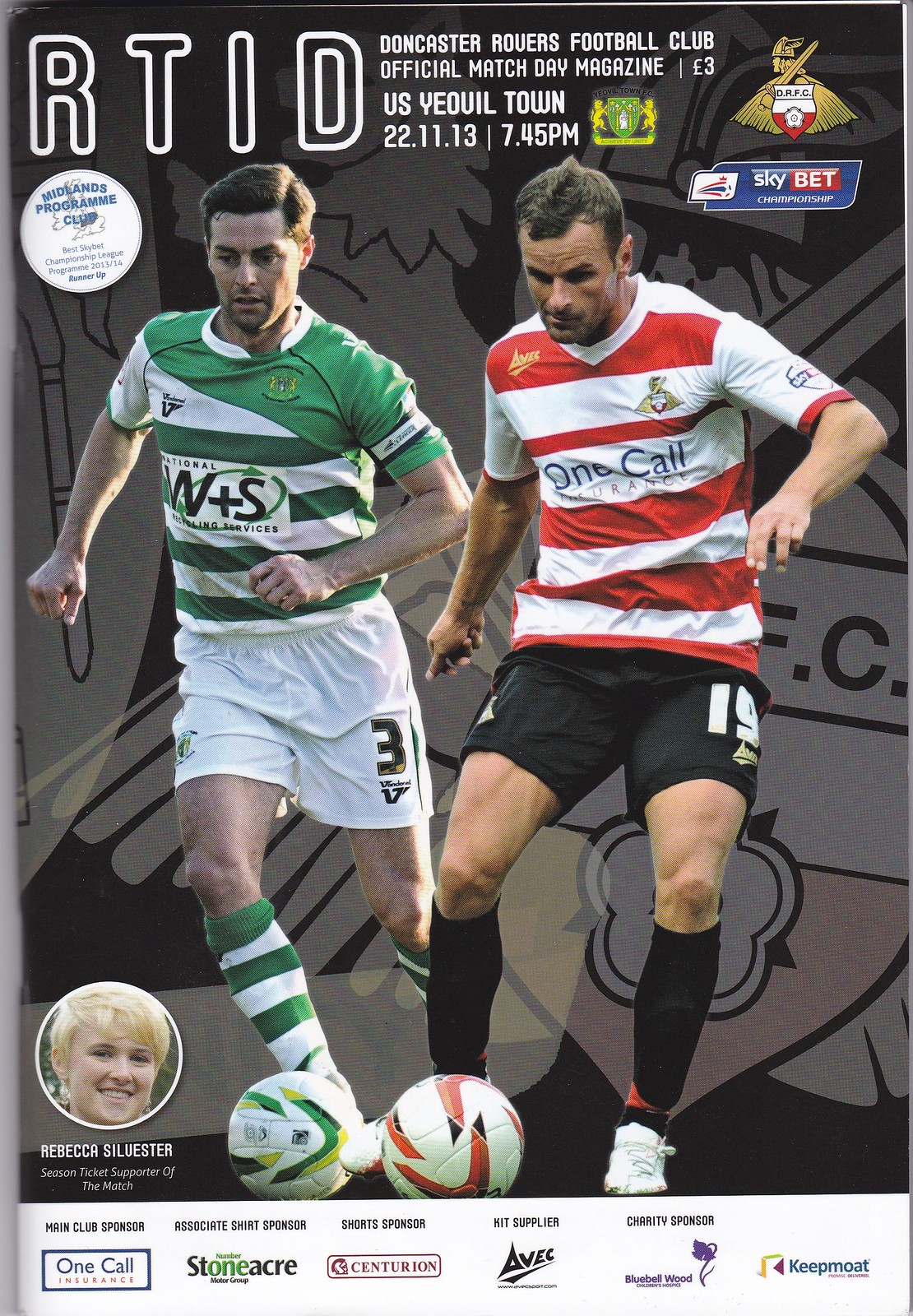The image is a color-printed cover of a soccer program for the Doncaster Rovers Football Club official match day magazine, dated 22-11-13 at 7.45pm. At the top in bold white text, it reads "RTID." The background is a black and grey design featuring the football club's logo. The main focus is on two soccer players facing the viewer in a dynamic running position, each dribbling a ball that reflects their team colors. The player on the left is wearing a green and white striped jersey with white shorts, marked with the number three in black, and green and white striped socks. This player, with dark hair and clean-shaven, is dribbling a soccer ball with a green and yellow pattern. The player on the right sports a red and white striped jersey with black shorts featuring the number 19 in white, black socks, stubble on his face, and is dribbling a ball with a reddish and black design. At the bottom left of the cover, there is a headshot of a smiling woman with blonde hair inside a circle, identified as Rebecca Sylvester, the season ticket supporter of the match. Below this, a white banner showcases various sponsor logos.